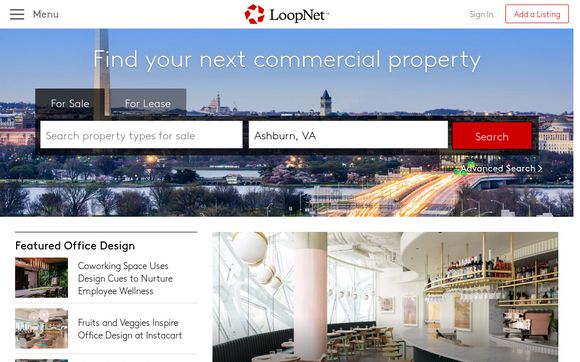This landscape-oriented screenshot features the LoopNet logo, identifying the website as a prominent real estate platform, located in the upper right-hand corner. Just below the logo is a red button labeled "Add a Listing". The main content section beneath it showcases a cityscape on a clear, blue-sky day, with a river running through the scene. At the top left of this section, there are two prominently displayed tabs: "For Sale" and "For Lease". Below the tabs is a search bar with the placeholder text "Search Property Types for Sale Ashburn, Virginia", accompanied by a red "Search" button and a link to an "Advanced Search" option.

To the left side of the main content, there are two featured sections with titles that read "Design Co-Working Space Uses Design Cues to Nurture Employee Wellness" and "Fruits and Veggies Inspire Office Design at Instacart", each accompanied by relevant images. The continuation of content is hinted at by the visible tip of another image peeking out from the bottom left corner, suggesting more information available upon scrolling.

On the right side of the screenshot, a large image of a modern-looking cafeteria or bar area is displayed, featuring sleek and stylish decor, indicating an ideal property that might interest potential commercial real estate buyers.